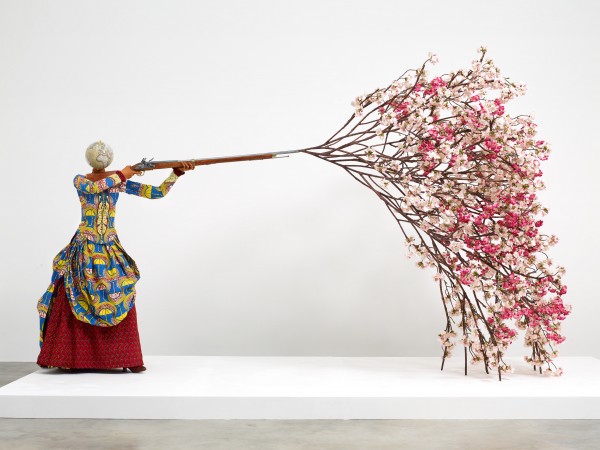The image depicts an intricate art installation featuring a faceless mannequin sculpted to resemble a woman. She stands on a modest white rectangular platform against a plain white wall, dressed in a vibrant, multicolored gown showcasing a lively mix of blue, yellow, and red hues. This outer garment, which extends down to her knees, is layered over a striking red skirt that drapes all the way to her burgundy heels. The mannequin's head is a featureless, globe-like sphere.

In a dramatic pose, the mannequin clutches an antique flintlock rifle, holding it as if to fire. Instead of a bullet, however, the rifle's barrel bursts into a cascade of delicate pink and white cherry blossoms, presented on intricate tree branches that appear to be organically growing out of the gun. This juxtaposition of violence and beauty forms a compelling visual narrative, seamlessly blending themes of life, death, and transformation within the confined space of the platform.